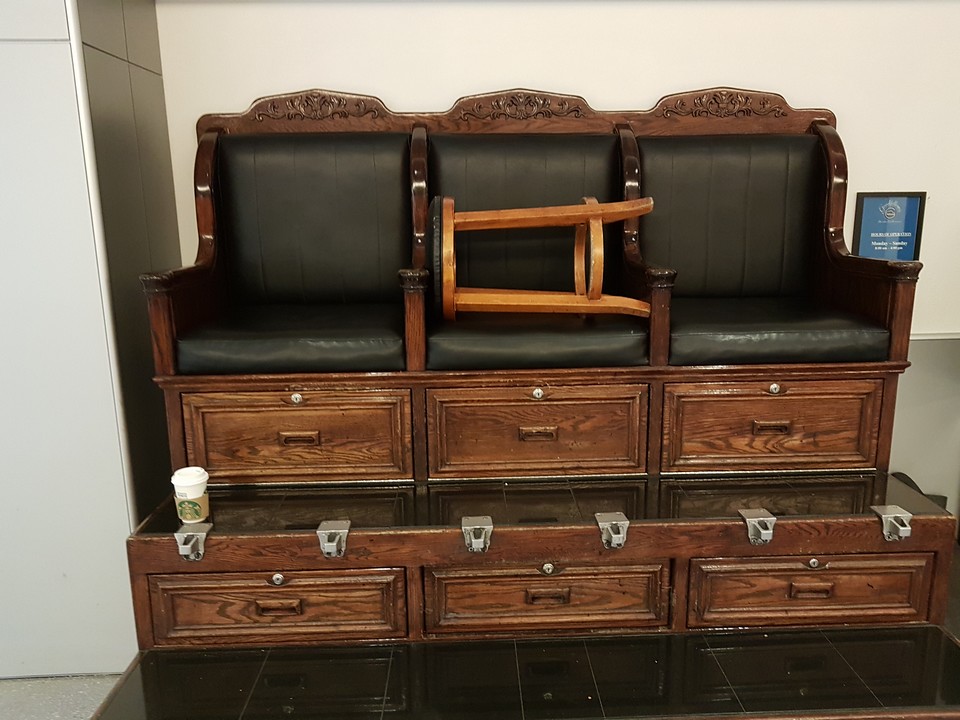This photograph captures an antique shoeshine seating arrangement, consisting of three connected black leather chairs, each with back and seat cushions, housed within a meticulously crafted wooden cabinet. The wooden structure incorporates a double deck of drawers beneath each chair, arranged in two rows. The chairs are separated and framed by ornate woodwork, including the arms of each chair. Elevated from the ground, the base features metal footrests in front of each seat, allowing clients to comfortably position their feet for shining.

A black-topped, round brown stool, used by the shoeshiner, is stored sideways on the middle chair. The cabinetry design is emphasized by the wood trim around the chairs and drawers, enhancing the antique aesthetic. Additional details include a white wall behind the setup, a side wall on the left, and a white Starbucks cup placed on the ledge to the left of the image. A shiny black floor contrasts with the intricate wooden furniture, and a blue sign in a black frame is visible to the right, though its text is illegible.